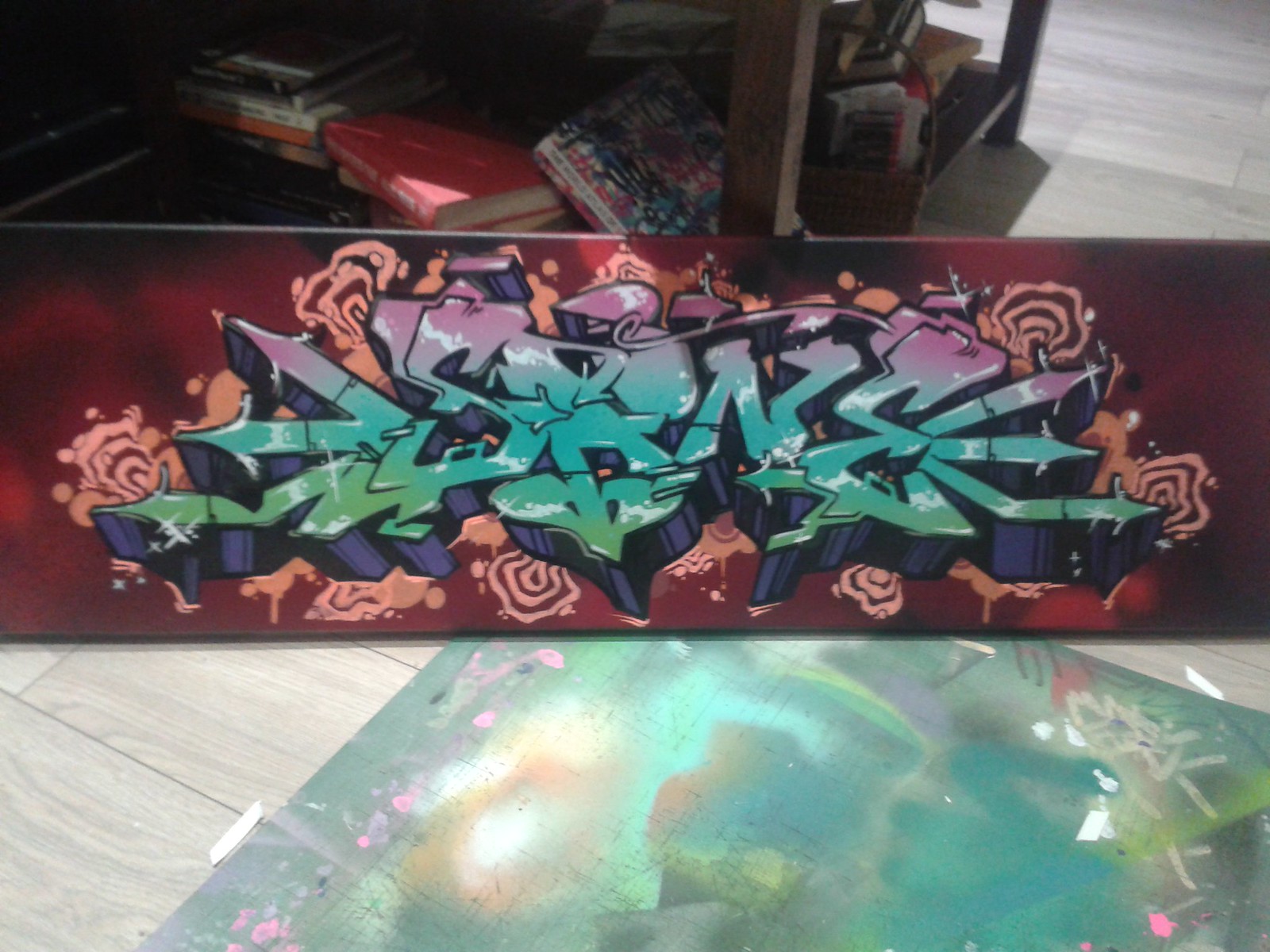The image features a rectangular painting with stylized graffiti letters, prominently displaying an abstract, dynamic three-dimensional style. The letters, mainly in green, aqua, purple, and pink, spell out "S-R-N-E" against a dark red and black background with orange swirls interspersed among them. The artwork, resembling the underside of a skateboard, is positioned indoors on a tan plank floor, elevated on a wooden stand with legs. Surrounding the painting, there is a wooden shelf, and a coffee table cluttered with a haphazard pile of books and a basket filled with more books. Additionally, in front of the primary painting, another green, abstract graffiti piece appears to be in progress.